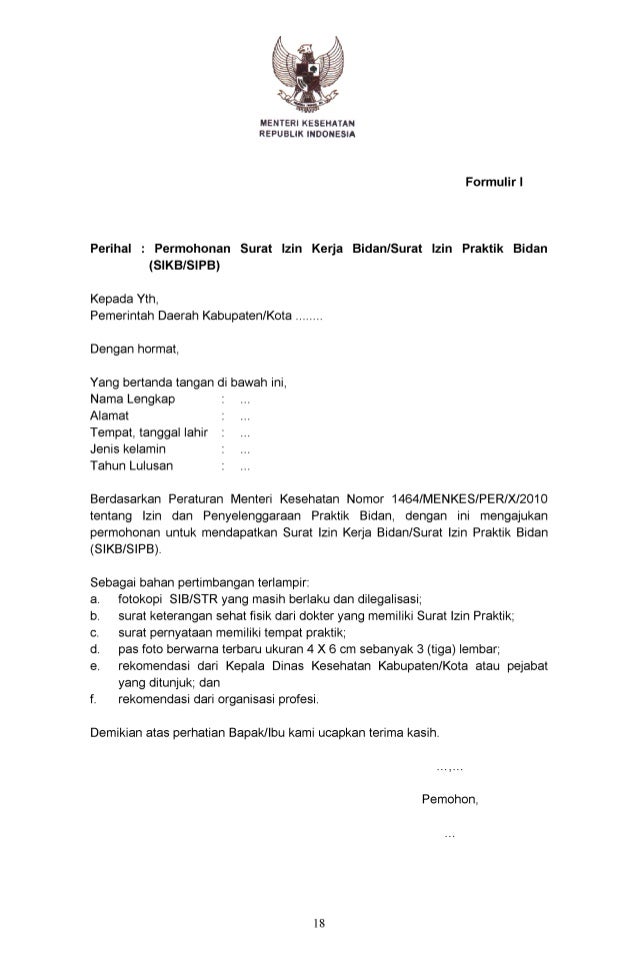The image is a black and white document, possibly a form or report, written in a foreign language. At the top of the document, there is an intricate letterhead featuring a stylized eagle emblem with its wings spread upward, which is clutching items in its claws and has a shield on its chest. Underneath the emblem, there are words including "Republic Indonesia" and possibly "Mentor." The body of the document contains multiple sections. There is a heading on approximately the fourth line, followed by a column of text and punctuation marks. Below this column, there are paragraphs of text, some labeled with letters A, B, C, D, E, and F. Towards the end of the document, there is a final sentence and a closing signature. Centered at the very bottom of the image is the number 18.